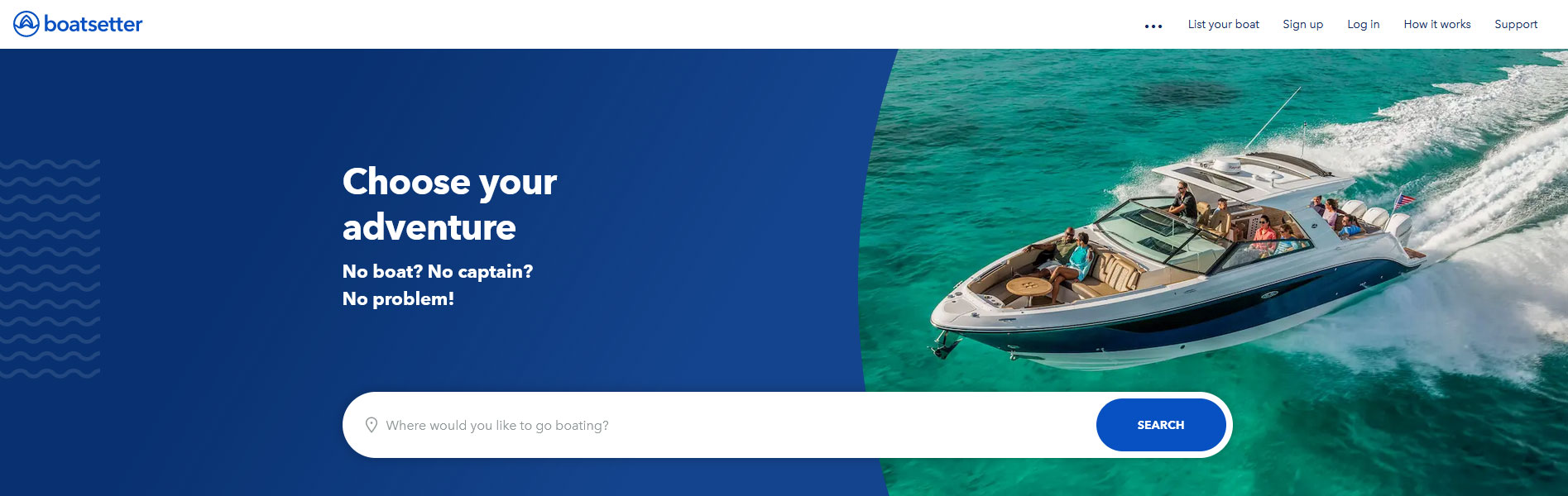This screenshot captures the homepage of a website named "Best Boat Setter." The top left corner features the site’s name accompanied by an icon resembling the prow of a boat emerging from the water, reminiscent of the iconic scene from "Jaws."

At the top right, the navigation bar lists several options from left to right: a horizontal three-dot menu, "List Your Boat," "Sign Up," "Log In," "How It Works," and "Support." Centrally located on the screen, a prominent banner reads, "Choose Your Adventure - No Boat? No Captain? No Problem." Beneath this, a search bar invites users to type in their desired boating location, with a blue search button positioned to the right of the bar.

The right side of the screenshot features an image depicting nine people aboard a two-story boat, leisurely enjoying their time on the water. This vibrant image adds a visual appeal, capturing the essence of the boating experiences offered by the website.